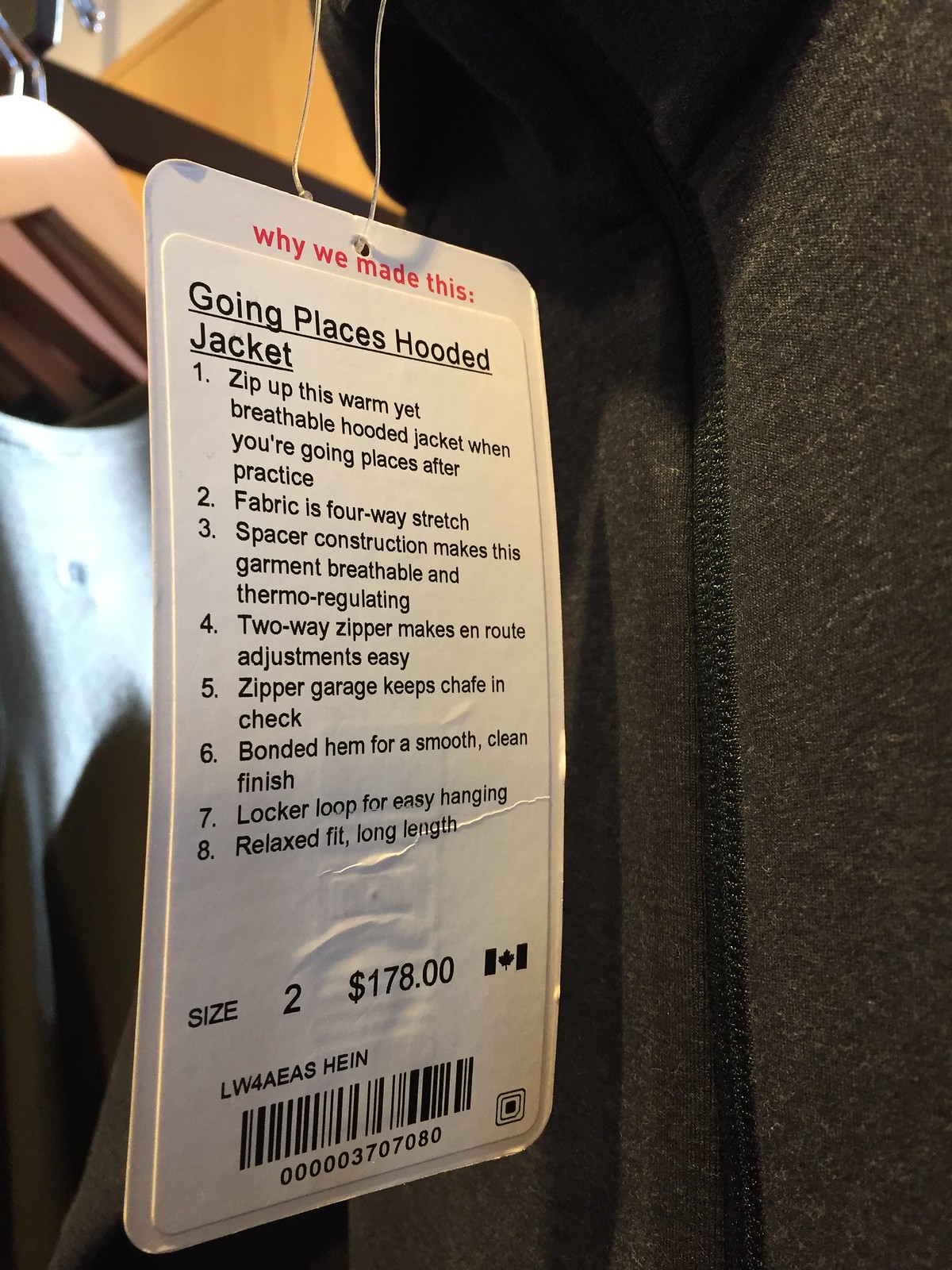This image depicts a dark gray zip-up jacket with a hood. A tag is prominently attached to the garment via a string. The tag features the heading "Why We Made This" in red and showcases detailed features of the "Going Places Hooded Jacket." Key attributes include: 
1. A warm yet breathable fabric ideal for post-practice wear.
2. Four-way stretch material.
3. Spacer construction for breathability and thermo-regulation.
4. A two-way zipper for easy adjustments.
5. A zipper garage to prevent chafing.
6. A bonded hem for a smooth, clean finish.
7. A locker loop for convenient hanging.
8. A relaxed fit with a long length. 

The jacket is a size 2 and is priced at $178, with a Canadian flag logo near the price. Additionally, there is a barcode at the bottom of the tag, with the number sequence "0003707080" and the caption "LW4EA SHE IN."